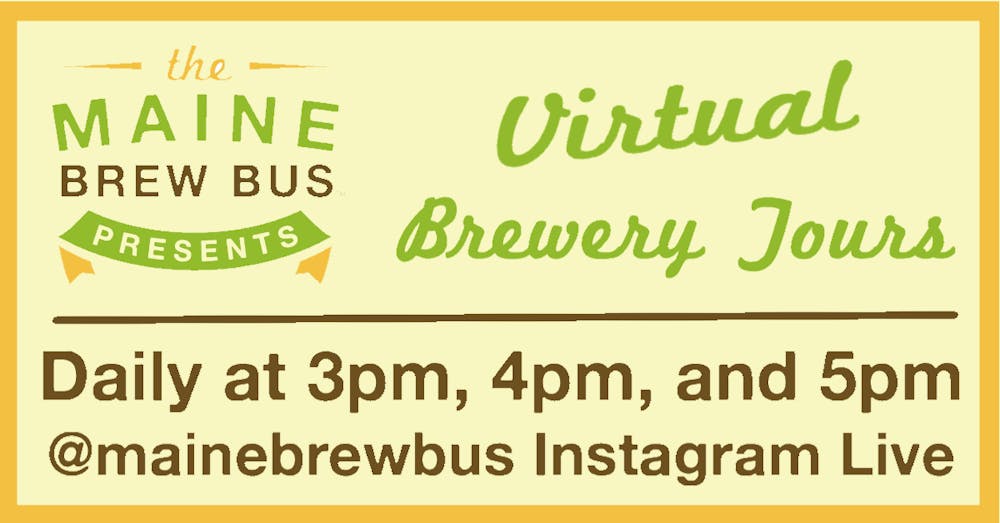The image is a detailed advertisement for virtual brewery tours presented by Maine Brew Bus, designed for social media platforms like Facebook or Instagram. The ad features a yellow background with an orange border, giving it a vibrant look. At the top, the text "The Maine Brew Bus Presents" is prominently displayed with "The" and "Brew Bus" in dark brown letters, while "Maine," in all caps, is written in green letters. Below this, in the center of the ad, the phrase "Virtual Brewery Tours" is also in green, with "Virtual" styled in a script font at an angle. A dark brown dividing line separates the main text from additional details at the bottom. Underneath this line, the ad specifies "Daily at 3 p.m., 4 p.m., and 5 p.m." in brown letters. Finally, the social media handle "@mainebrewbus" is noted, indicating that the tours can be accessed via Instagram Live.